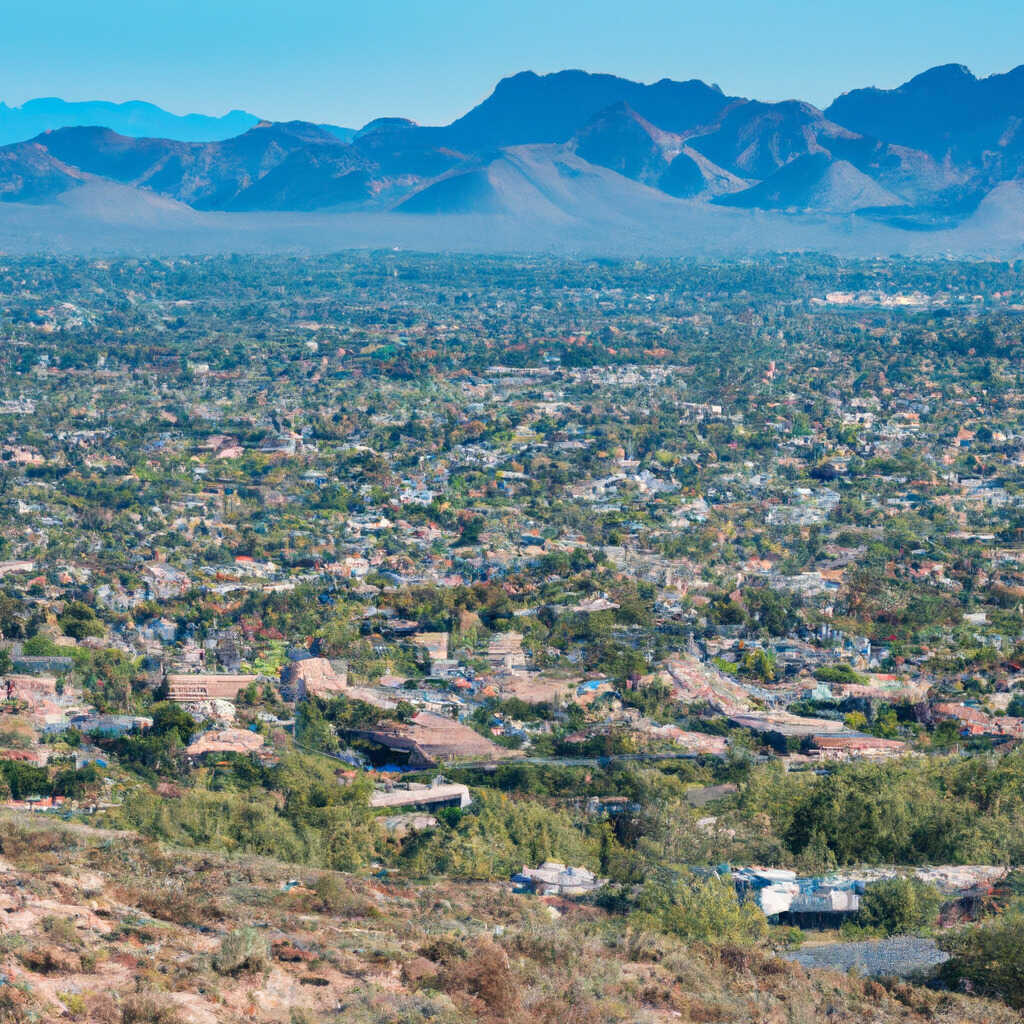The photograph captures a picturesque view of a suburban area, possibly somewhere like Salt Lake City, Utah or a similar locale. Taken from atop a hill or bluff, the scene overlooks a sprawling valley filled with numerous homes and small buildings, interspersed with lush green trees and shrubs. The foreground displays a scrubby hillside with sagebrush and other native plants, reflecting the arid, desert-like terrain. The valley stretches far and wide, showcasing a blend of light brown, sandy, and few red and white roofed buildings, set against a backdrop of smooth, dusty brown mountains. The day is bright and clear, with a blue, midday sky illuminating the landscape. Despite the development, the area retains a significant amount of greenery, giving it a grassy, almost rural feel. In the distance, a layer of smog lingers below another set of towering mountains, adding depth to the vast, natural scenery.